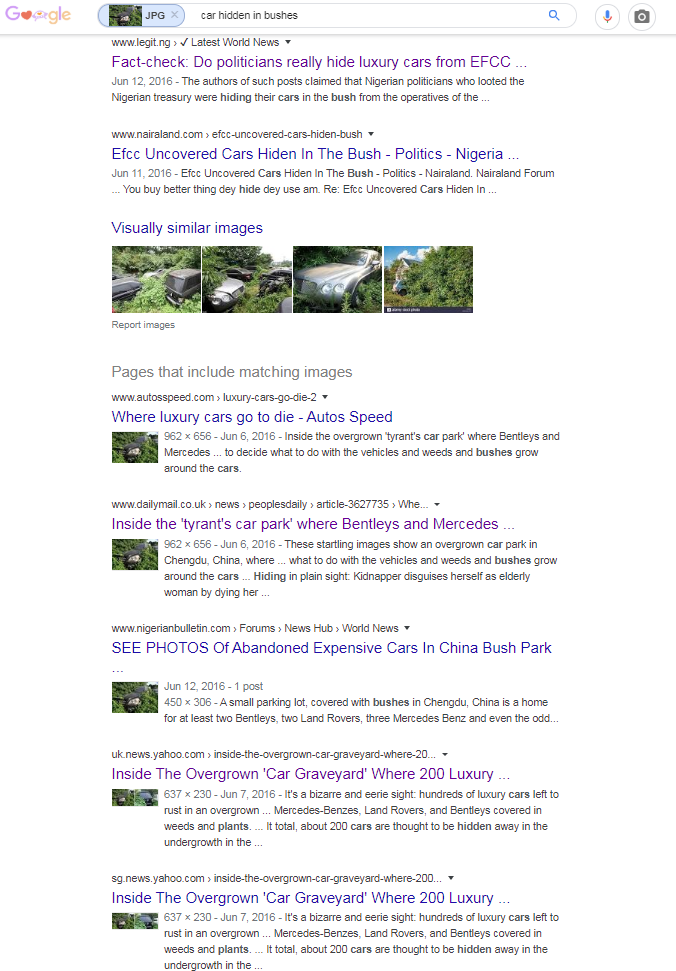A Google search results page is displayed on a special themed day, likely Valentine's Day, indicated by the first "O" in the Google logo being replaced with a red heart. Positioned centrally on the page is the Google search bar, into which the phrase "car hidden in bushes" has been entered. The user has clicked the magnifying glass icon to initiate the search. Above the search bar, there are additional icons for voice search and image search, represented by a microphone and a camera, respectively. The search results display two advertisements at the top, followed by a set of four images depicting cars obscured by bushes. Below these images, snippets of webpages containing matching visuals are listed.